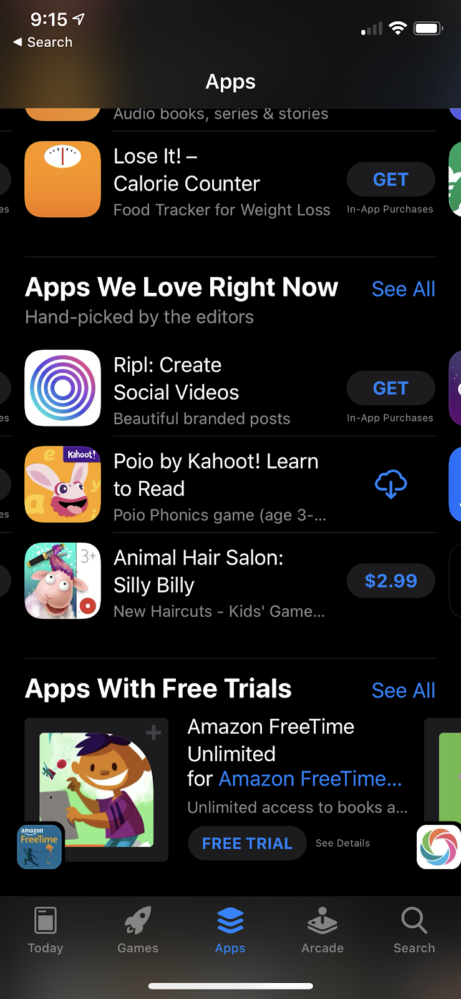A screenshot of a smartphone screen with a black background showing the time as 9:15. The signal strength indicator shows a single bar, signifying weak cellular reception, while the battery indicator displays robust charge level. The search bar at the top indicates an ongoing search for apps. Below, a list of apps is partially visible. The first app listed is "Audiobooks, Series, and Stories," followed by "Lose It! – Calorie Counter," a food tracker for weight loss with an orange scale logo. 

Further down, there's a section titled "Apps We Love Right Now," curated by editors. It features "Ripple – Create Social Videos," identifiable by a logo with multicolored concentric circles, and "Poi," an app characterized by its giant bunny rabbit icon on an orange background. 

Other apps include "Kahoot! Learn to Read – Polo Phonics Game," which can be downloaded, and "Animal Hair Salon – Silly Billy," priced at $2.99, featuring kids' games with new haircut options. 

There's also a category for "Apps With Free Trials," highlighting "Amazon FreeTime Unlimited," depicted by an image of a child playing and offering a free trial. At the bottom navigation, icons for "Today," "Games," "Apps," "Arcade," and "Search" are visible.